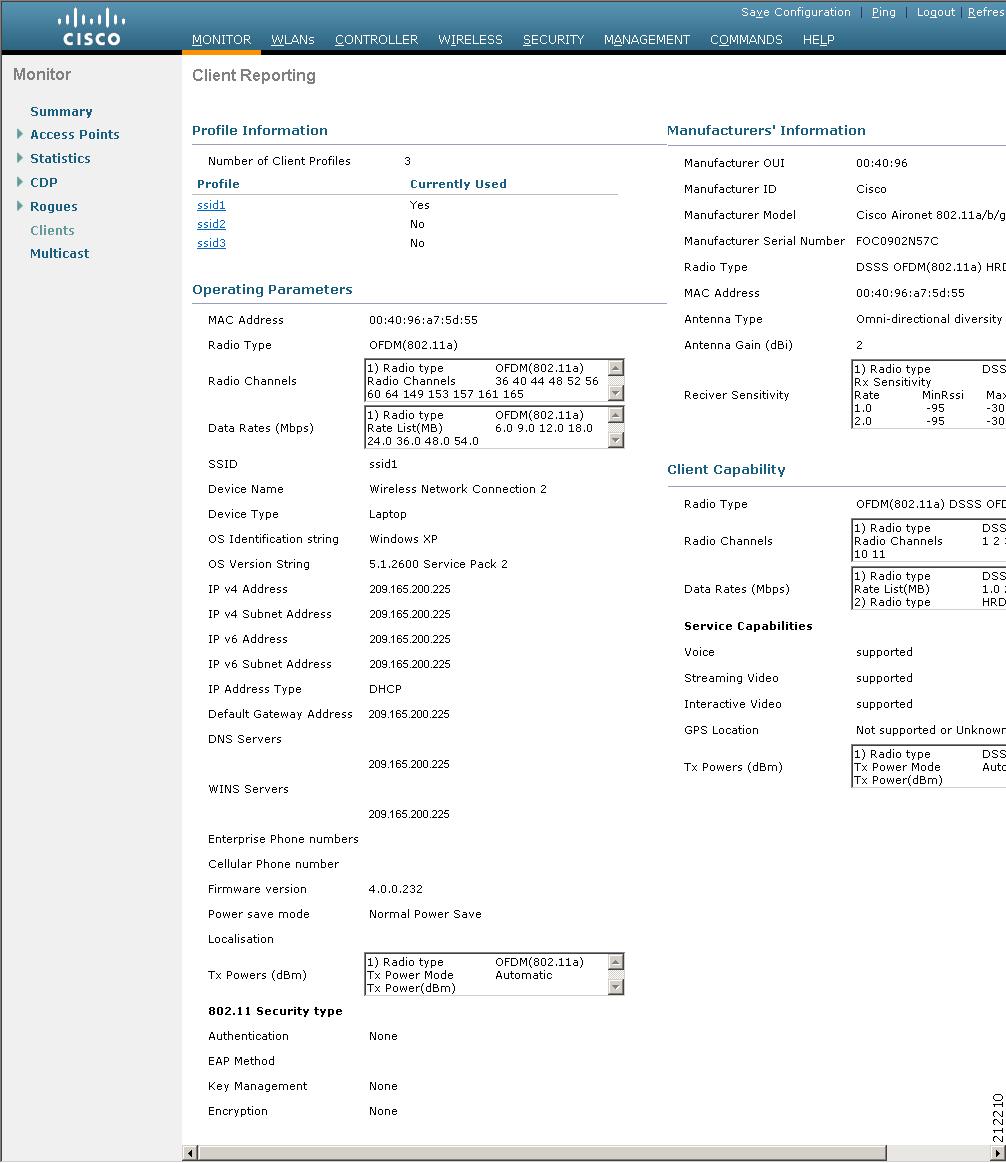**Image Caption: Detailed Breakdown of Cisco Network Monitoring Dashboard**

At the very top of the image, the Cisco Network Monitoring Dashboard is displayed, featuring tabs for Monitor, WLANs, Controller, Wireless, Security, Management, and Commands. The options above the dashboard include safe configuration, ping, logout, refresh, various licenses, monitors, summary, access points, statistics, CDP (Cisco Discovery Protocol), rogues, clients, and multicast.

In the center section, there's detailed client reporting information. This includes profile information with the number of client profiles, profile SSIDs labeled as SSID1, SSID2, and SSID3, indicating whether they are currently in use (yes for SSID1, no for SSID2 and SSID3). It also displays operating parameters such as MAC addresses, radio time, channels, data rates, SSIDs, device names, device numbers, other certification strings, address types, process modes, localization, 2x power, and 802.11 standards. Security type, security management, and encryption details are also specified.

On the top right, my virtual machine interface is shown. It includes Touch ID, Cisco's physical model and internet infrastructure, serial number, radio time, MAC address, antenna gain, receiver sensitivity, client capability, radio time, radio channel, data rates, and VPS. 

The comprehensive layout provides a thorough overview of the network's configuration and performance metrics essential for effective network management.